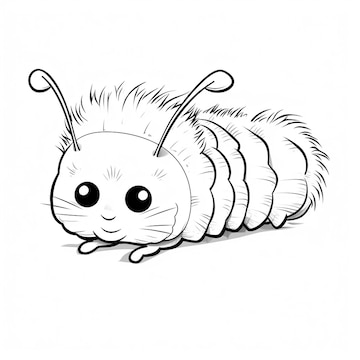This black and white image depicts a stylized caterpillar-like creature rendered in a simple, cartoonish line drawing. The overall shape of the drawing is rectangular, with the top and bottom sides being twice as long as the left and right sides, suggesting a landscape orientation. The caterpillar, appearing to crawl towards the left, features a segmented, furry body with small nubs instead of legs, giving it an intriguing, unique movement style. Its face is endearing and human-like, characterized by round, beady eyes, two chins, and a smiling mouth with pouty lips. The facial expression is friendly and inviting. Prominently, the creature has two large antennae on either side of its forehead, ending in rounded bulbs, adding to its whimsical appearance. This detailed yet simple, text-free drawing captures the charm and cuteness of the caterpillar with its meticulous design elements.